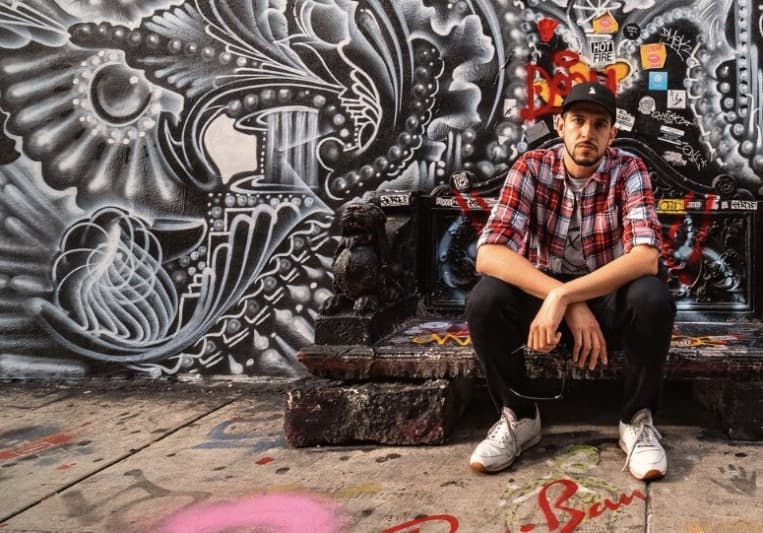This outdoor photographic image features a white man dressed in urban attire sitting and crouching on a sidewalk. He wears a red plaid shirt with sleeves pulled up to the elbows, a black graphic t-shirt underneath, black pants, white sneakers, and a black baseball cap. The man, who has a mustache and goatee, crosses his arms while looking directly at the camera. He is situated against a backdrop of a predominantly black and white graffiti mural with floral emblems around a central pillar, accented by some orange and red splotches. Notably, the words "Hot Fire" appear on a sticker affixed to the wall behind him, and the word "BAM" is painted in red on the sidewalk beneath his feet, which also features various other graffiti. The overall scene exudes an urban, street-art ambiance, with additional graffiti elements and stickers visible in the background.